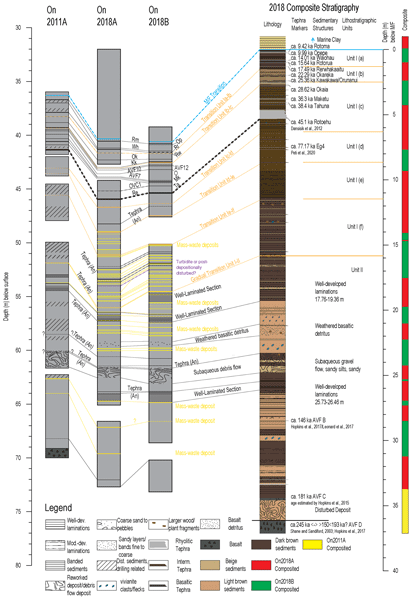The image is a detailed and complex diagram titled "2018 Composite Stratigraphy," with this title prominently displayed in bold text at the top right corner. This concept likely pertains to archaeology. On the left side, there is a vertical axis labeled from 80 at the bottom to 30 at the top, marked in increments of 5. Adjacent to this axis are three stratigraphic columns, each rendered in gray and labeled at the top as "2011 A," "2018 A," and "2018 B" from left to right. Additionally, a fourth stratigraphic column, distinguished by its various shades of brown, is located further right.

Each column is composed of different layers, resembling a geological cross-section, with numerous lines extending from these layers to a secondary graph on the right side of the image. These lines, carrying both text and coloring for differentiation, include black lines with black text, orange lines with orange text, and one dashed blue line with blue text. The bottom of the image features a legend that deciphers the various colors and designs used within the diagram, and there's also a color-coded vertical key positioned on the far right side.